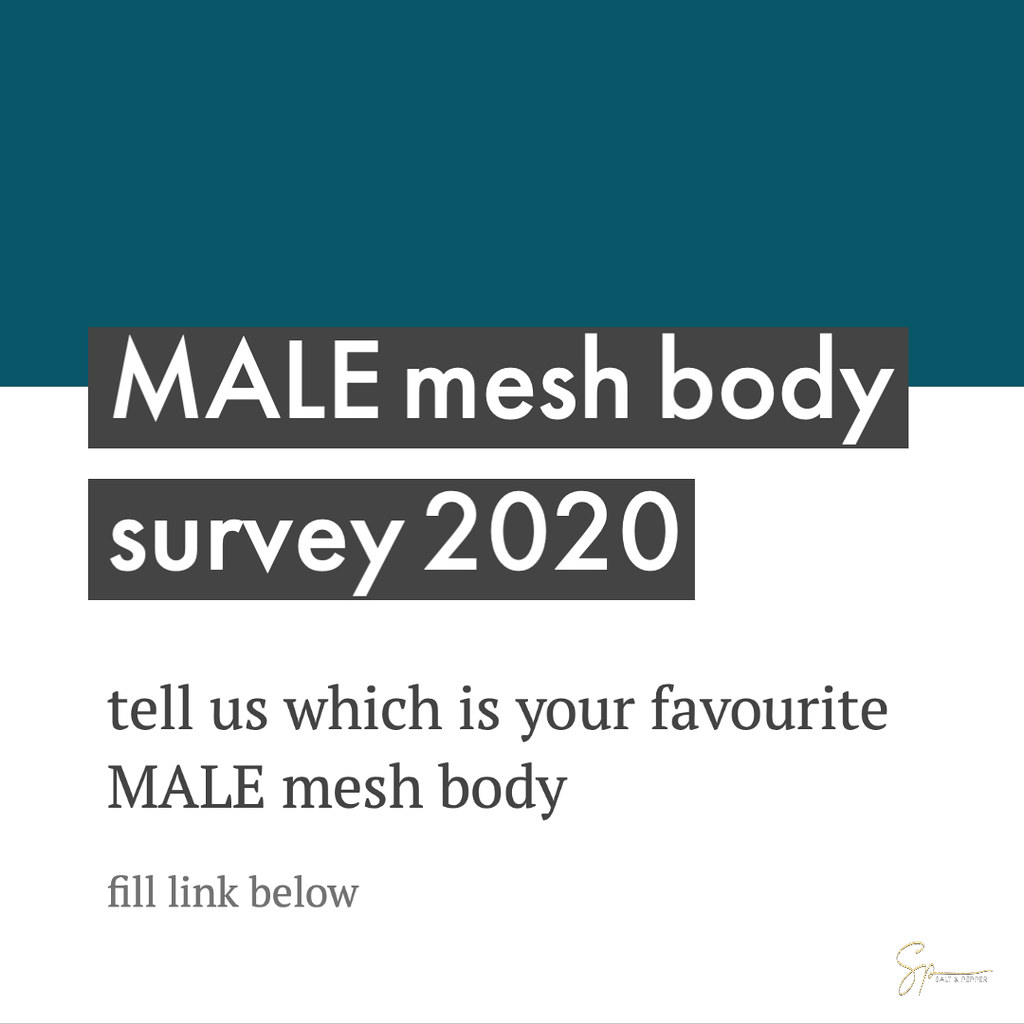The image is a square poster with a distinct division of colors and text. The top third features a dark blue block that fades into a dirtier blue, almost navy hue. Overlapping the bottom part of the blue block is a black rectangle with the words "MALE MESH BODY" in white, capitalized letters, though "male" is particularly prominent. Directly below this is another black rectangle, slightly larger, stating "survey 2020" in lower and uppercase white letters. Beneath these blocks, on a white background, is a line of text in black letters that reads, "Tell us which is your favorite male mesh body." Below this, in smaller, lighter gray letters, it says, "Fill link below." The lower right corner contains a small logo which is not clearly defined in the description. The design aims for a clean and straightforward look with minimal external boundaries.